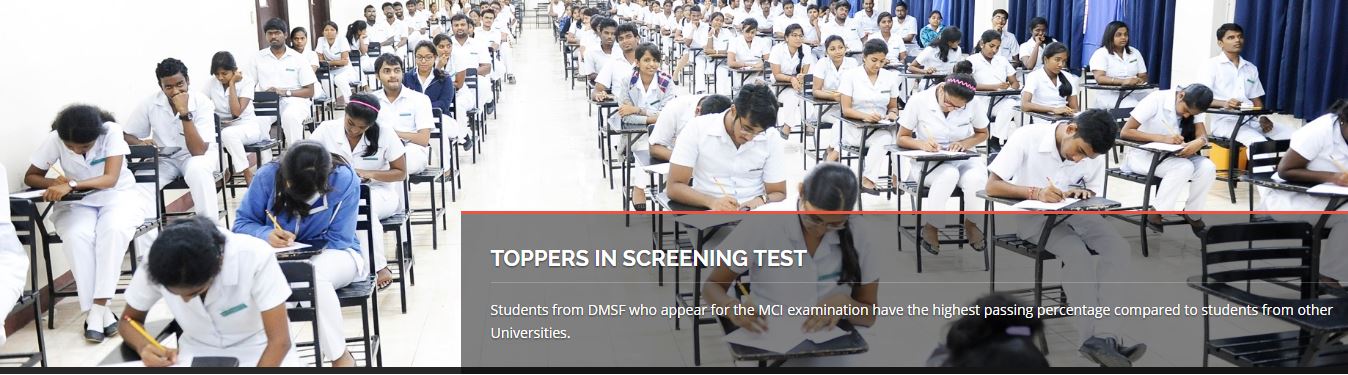The image appears to be an advertisement, possibly from a website, depicting a large group of students, likely from an Asian country given their ethnicity, taking an exam in a spacious indoor setting. The students, numbering between 50 to 100, are seated in long, seemingly endless rows of desks. They are all dressed in pristine white uniforms, complete with badges, suggestive of a possible medical profession. The solemn and focused expressions on their faces indicate the serious nature of the test they are taking. The room is characterized by its white and wood tan colors, with blue elements, such as curtains on the right-hand side. In the bottom right corner of the image, there is a text box with the headline "toppers in screening test" and additional smaller text that is partially legible, mentioning something about students at universities and comparing their high passing grades to other institutions. The overall scene is one of intense academic concentration, with the students absorbed in their exam papers.